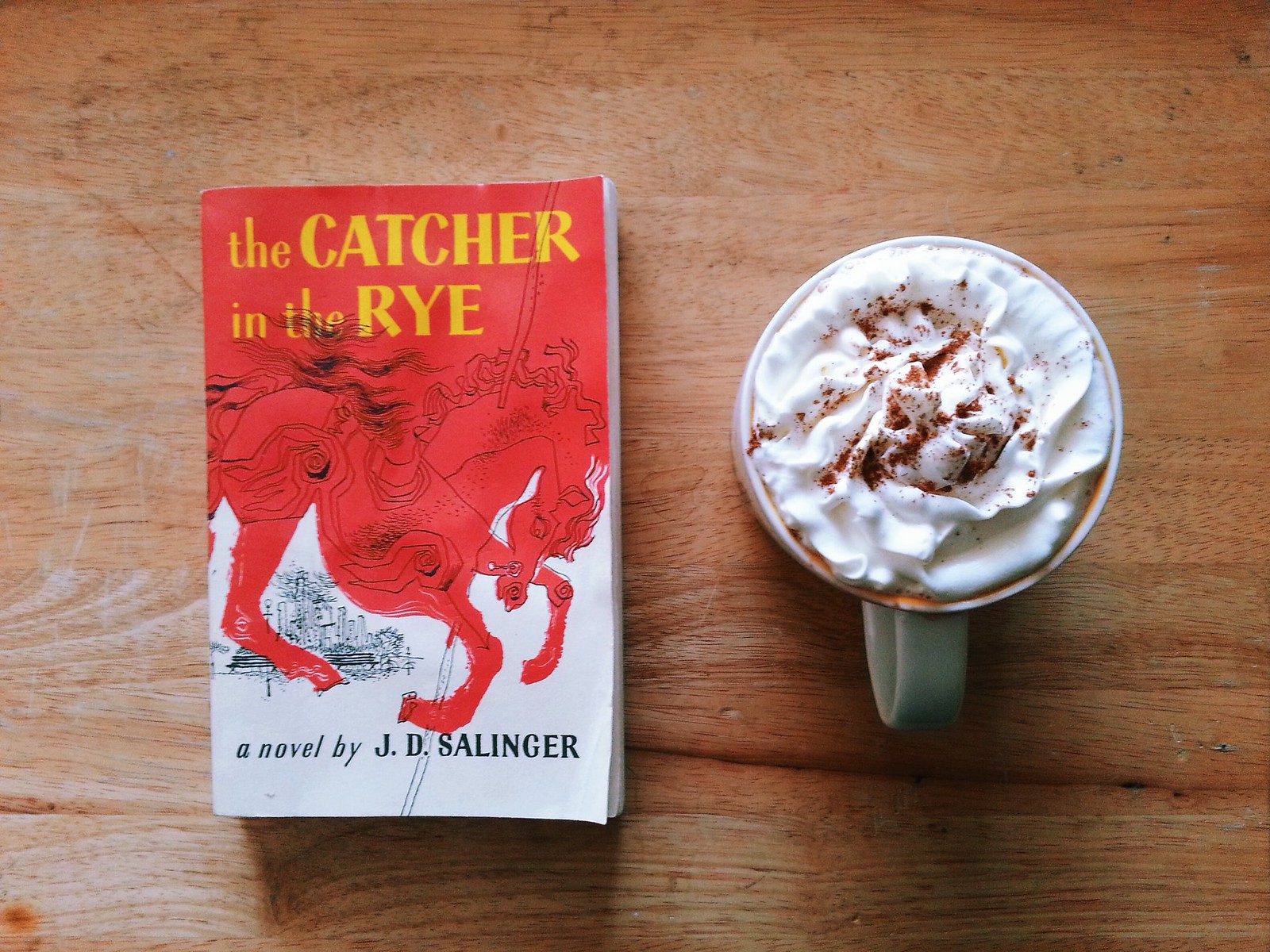The image is a bird's eye view of a wooden surface, likely a table, with two main objects positioned at the center. On the left lies a paperback copy of the book "The Catcher in the Rye" by J.D. Salinger. The book's cover features a red top section with a design that forms the shape of a horse, transitioning into a white bottom section. The title, "The Catcher in the Rye," is written in yellow at the top, with "a novel by J.D. Salinger" in black at the bottom. To the right of the book is a coffee cup, which is filled with a hot coffee drink topped with whipped cream and a sprinkle of what appears to be cinnamon. The handle of the cup, which is green, faces the bottom edge of the photograph. Both the book and the cup cast shadows on the table, adding depth to the composition. The image appears to be taken indoors, likely in a kitchen setting.